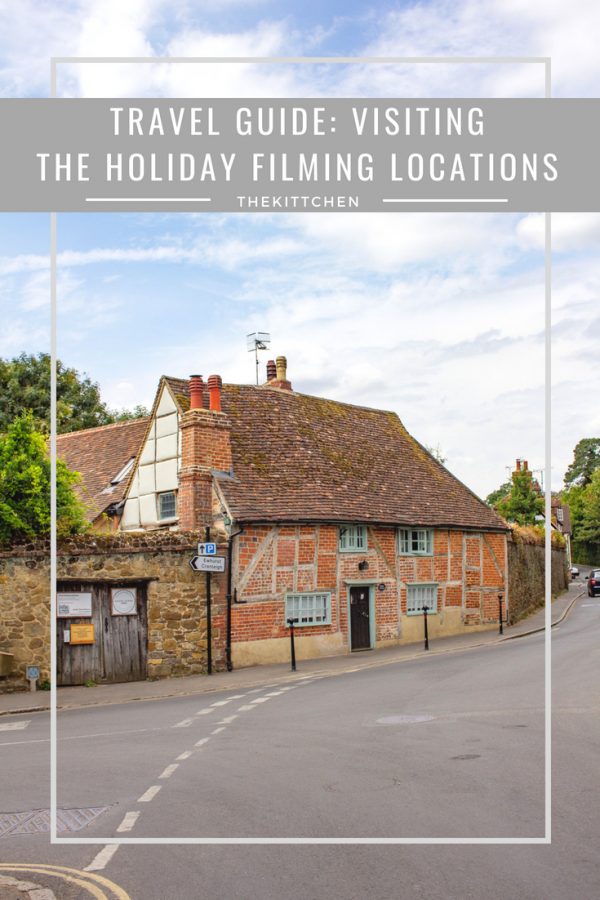This image is part of a travel guide titled "Visiting the Holiday Filming Locations: The Kitchen," with the words 'Holiday' and 'Locations' underlined and showcasing the text within a gray-bordered frame filled with white text. The image captures an old brick house on a well-kept road in an old British town, indicative by the parked car on the left side of the street. The red-brick structure features distinct gray-white outlines, four light blue-bordered windows, and a prominent brown door. Flanking the door are two windows on either side, with one more window above the door and another above the right-side window. The house has an A-shaped arc profile crowned with an old chimney featuring two exits. To the left of the house, additional doors are ensconced within the brick wall, each adorned with three various signs. The scene is further surrounded by gray borders along the edges, adding a neat framing to the travel guide image.